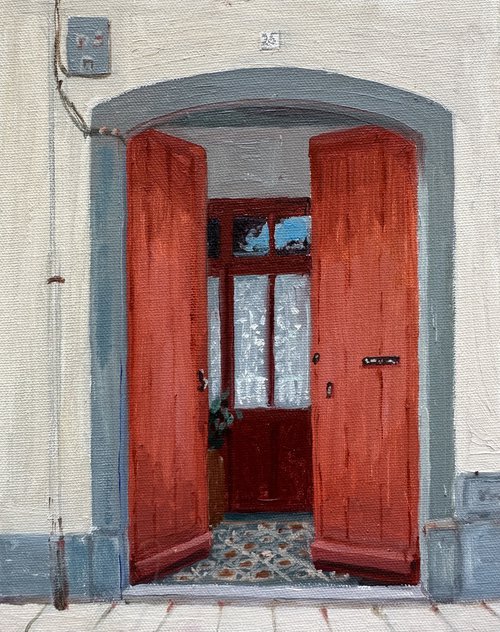This painting depicts the facade of a building with a distinct archway as its focal point. The structure features white siding, accented by blue baseboards and blue trim framing the arched doorway. Above the entrance, the number "25" is displayed on a small white square plaque. The double doors are crafted from rich redwood and are slightly ajar, revealing an internal set of doors that have glass windows. To the left of the entrance, a pipe ascends along the building's exterior, and an electrical box is mounted in the upper left corner.